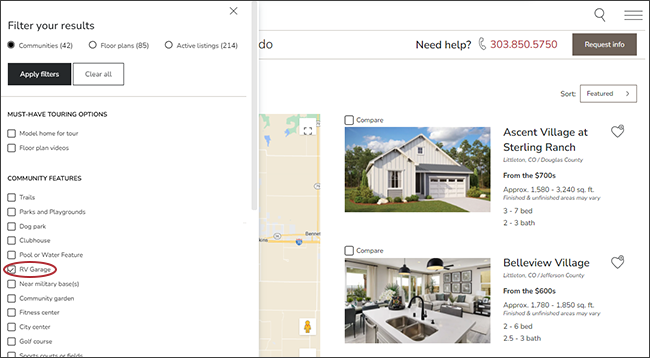The image displays a detailed user interface of a real estate application. It prominently features a "Filter Your Results" section, highlighting that there are 214 active listings available. The community is identified as having 42 units, with floors ranging up to 85. Options to "Apply Filters" and "Clear All" are visible, along with prompts for "Must Have Touring Options." For additional assistance, a contact number is provided: 303-850-570. The interface concludes with a polite message, "Thank you for watching."